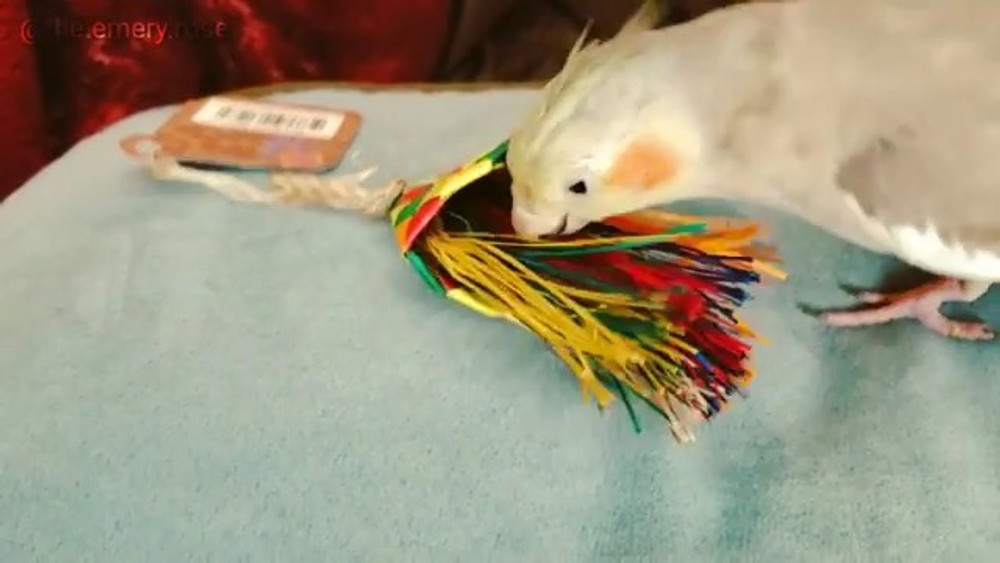The image depicts a somewhat blurry scene featuring a white parrot-like bird, likely a parakeet, emerging from the upper right corner of the frame. The bird's head, with a distinctive orange circular spot on its cheek and a small black eye, is turned downward toward a colorful tassel-like bird toy. This toy, reminiscent of a graduation cap tassel, boasts vibrant threads in red, yellow, green, blue, and brown, with an attached white cord and a cardboard tag bearing a UPC code. The bird appears to be interacting with—perhaps pecking at or dragging—this toy. Visible amid the multicolored threads is one of the bird's feet, characterized by three pointy claws. The setting seems to be an indoor space with a marbled gray and white surface, possibly a countertop, and a maroon curtain backdrop in the upper left side of the slightly out-of-focus image. An indistinct string of text, including an ampersand, overlays the top left corner, possibly indicating a website, although it blends into the curtain and remains unreadable.